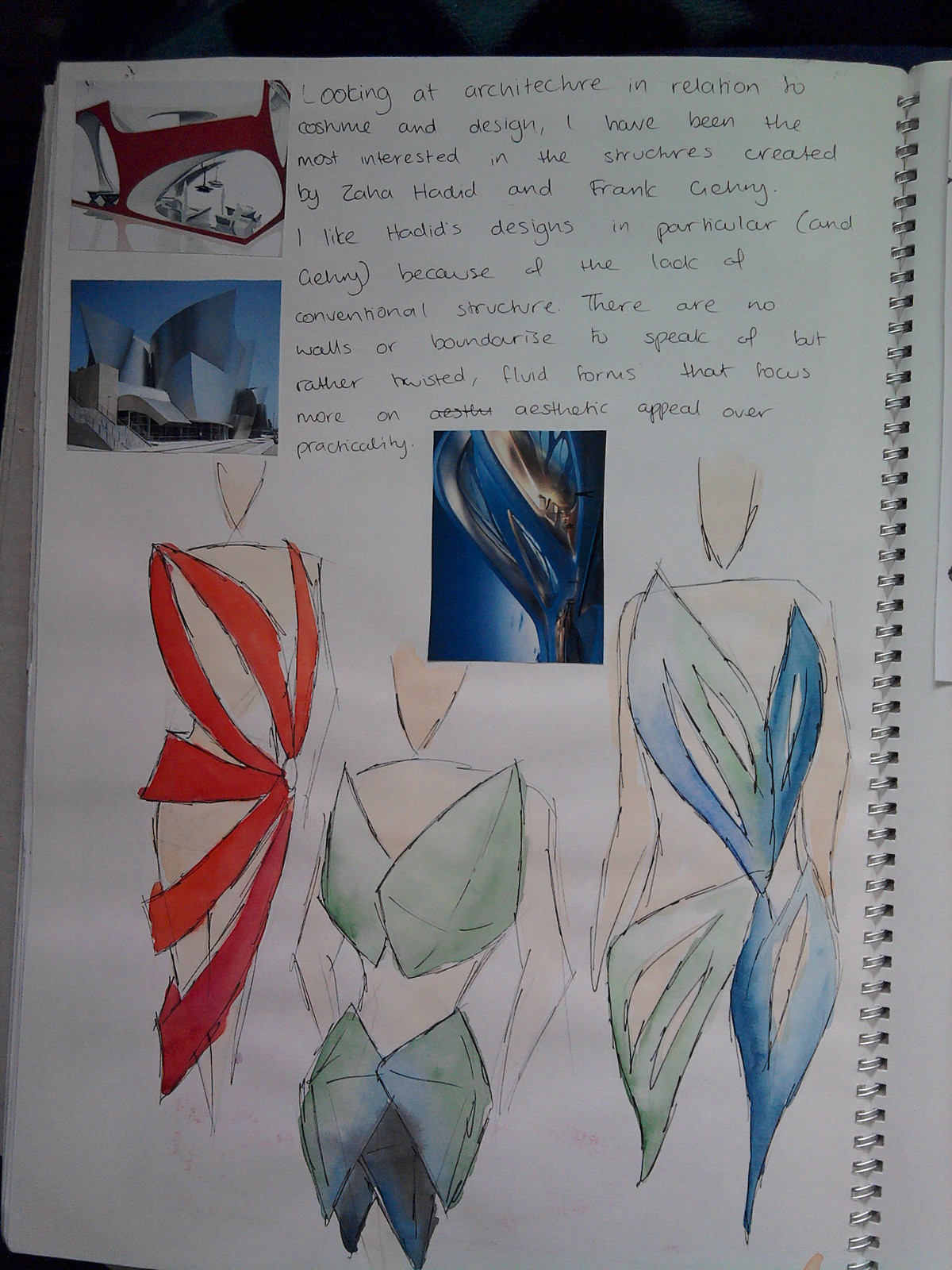This image depicts a page from an art student's notebook, highlighting a synthesis of architectural and fashion design. The lower section features three intricately drawn designs of women wearing dresses, likely inspired by the architectural concepts. At the top left corner, there are two overlapping photographs of sculptures. Another sculpture is prominently positioned in the middle of the page. The handwritten note, in cursive, reads: 

"Looking at architecture in relation to costume and design, I have been the most interested in the structures created by Zaha Hadid and Frank Gehry. I like Hadid's design in particular and Gehry's because of the unconventional structure. There are no walls or boundaries to speak of, but rather twisted, fluid forms. It's more an aesthetic appeal over practicality."

This artistic endeavor combines detailed sketches, possible watercolor coloring, and collaged images to explore the dynamic interplay between architectural forms and fashion design, embodying a creative and scholarly approach to design studies.